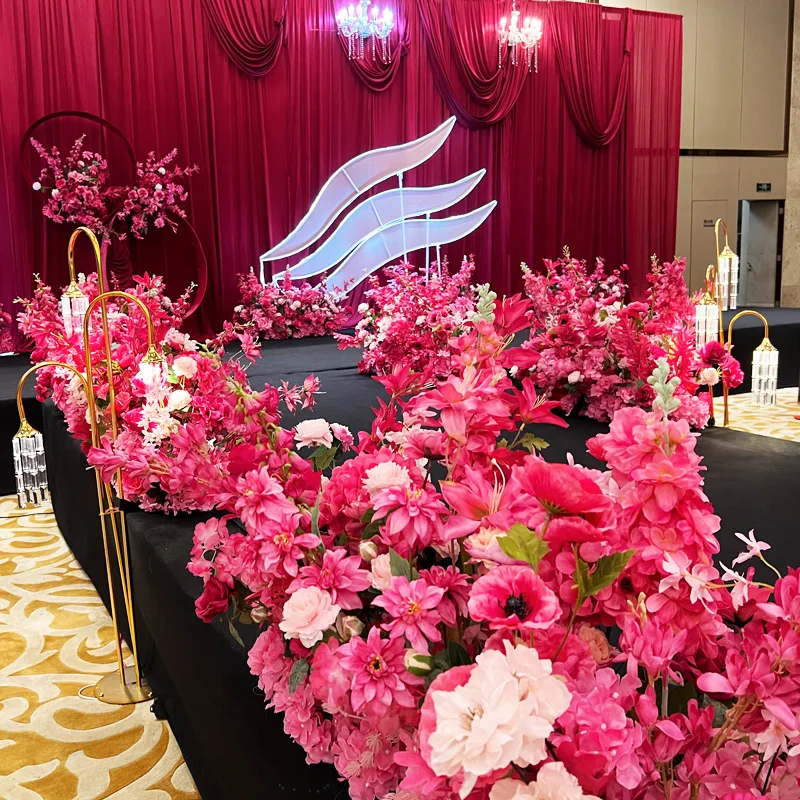The image captures a very elaborate and ornate wedding backdrop dominated by rich, scarlet red drapery. The foreground is a lush display of pink, red, and white flowers, predominantly roses, arranged in meticulously garnished bouquets that also include various types of ornate flowers. In the background, a stage or runway is set with a black rug, framed by large red curtains that add a dramatic flair to the scene. Adorning the sides of the room are brass curved stands holding golden lamps, while elegant candelabras hang from the ceiling, casting a warm glow over the setting.

A white logo resembling three waves is visible on the backdrop, adding a touch of modernity to the classic decor. The tables present are draped in black tablecloths and are lavishly adorned with large bouquets of roses, enhancing the luxurious and celebratory atmosphere. There are no people or textual elements in the image, allowing the viewer to fully appreciate the intricate details and sumptuous ambiance of the wedding display. The entire scene is brightly lit, contributing to a very clear and visually captivating image.